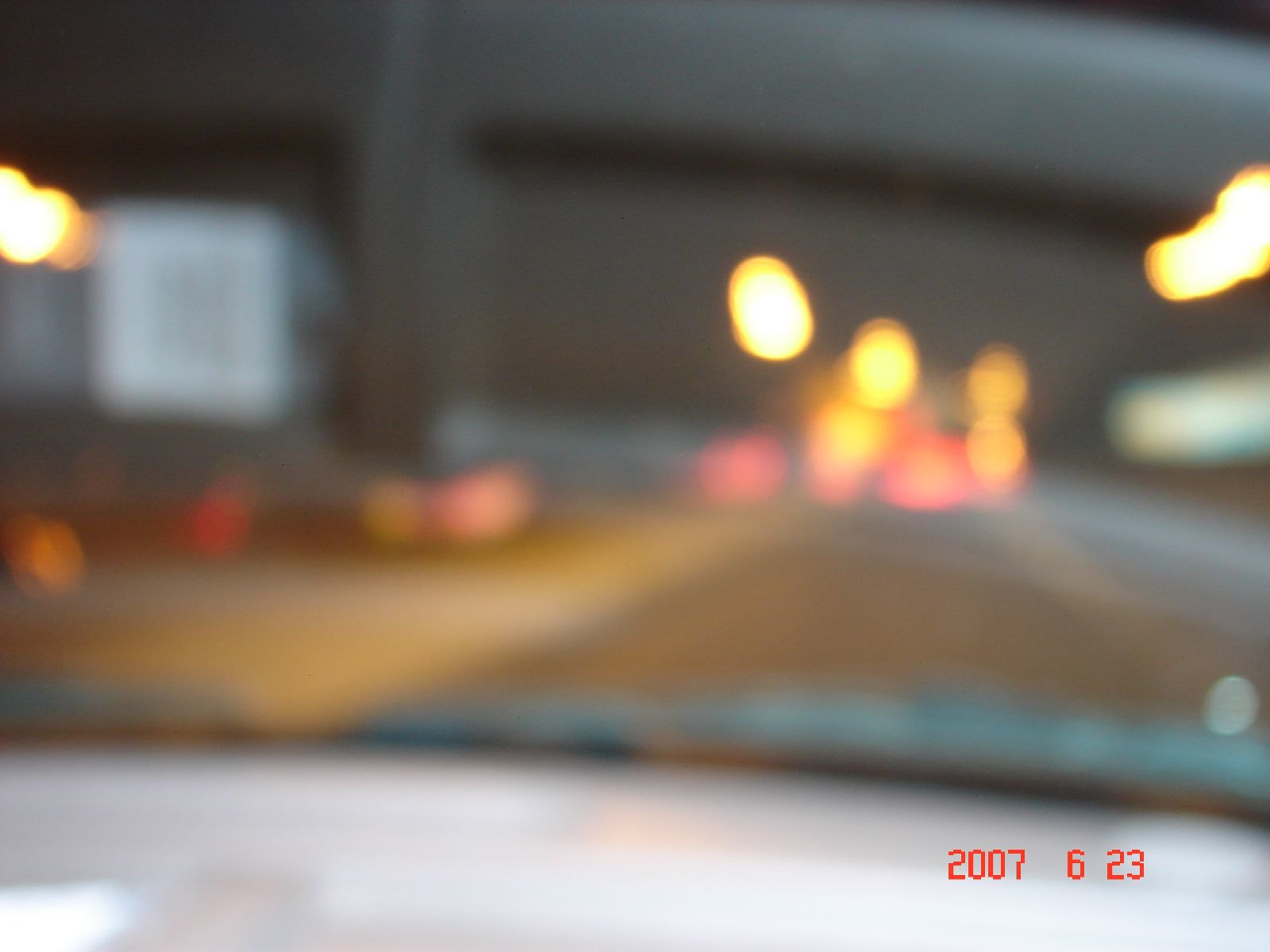A very blurry photograph appears to be taken from inside a vehicle, likely through the windshield. The top three-quarters of the image are dominated by the windshield, while the bottom quarter shows a white area that may be the dashboard. Between the windshield and the dashboard, some blurry windshield wipers are vaguely visible. The scene outside suggests nighttime, as the upper part of the picture is dark, punctuated by dim street lights and various vehicle lights. Ahead, several red lights, likely from cars, and yellow lights stand out in the darkness. To the far left, a large white square, possibly the back of a truck, can be discerned. At the bottom right corner, a timestamp in red reads "2007 6 23," indicating the date the photograph was taken.